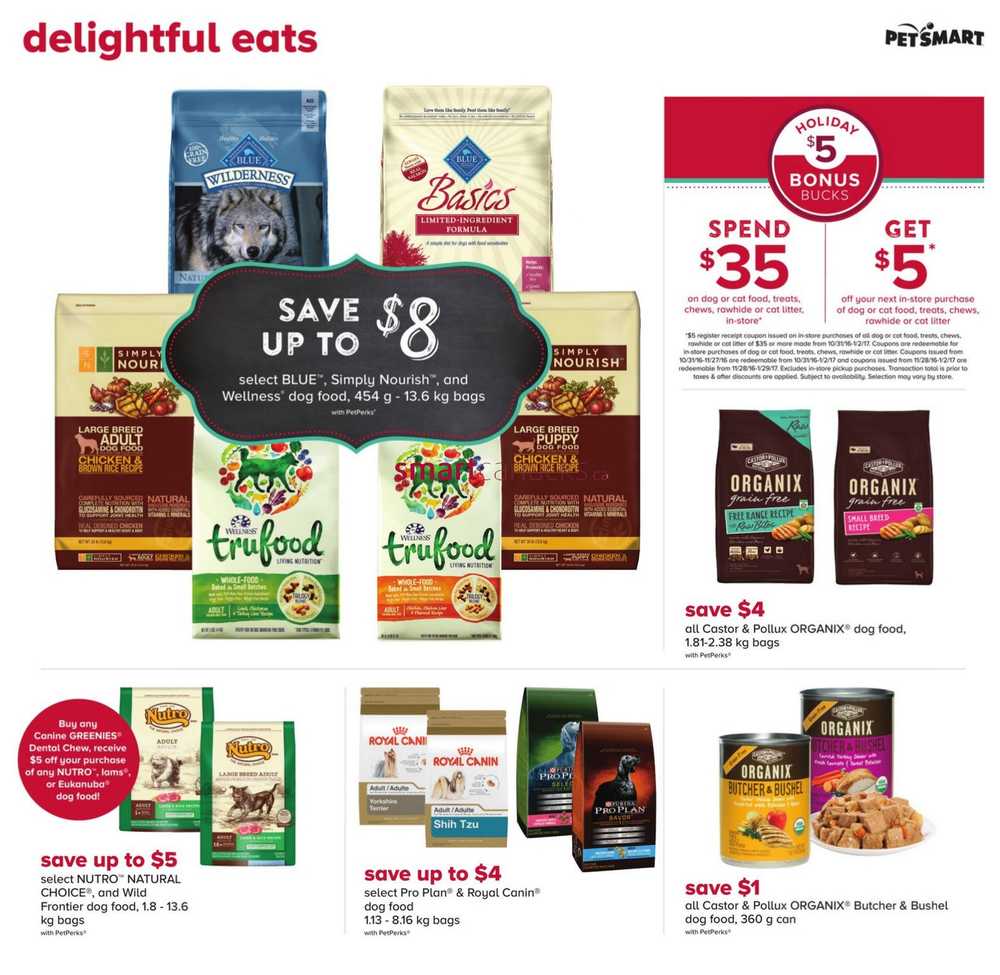This photograph showcases an array of premium dog food products available at PetSmart, detailed with various promotional offers. At the forefront, there's an enticing deal to save up to $8 on select Blue, Simply Nourish, and Wellness dog food, available in both 454 grams and 3.6 kilogram bags. These options cater to both puppies and adult dogs, ensuring balanced nutrition for different life stages. 

Below this, another promotion offers up to $5 savings on select Neutro, Natural Choice, and Wild Frontier dog food, ranging from 1.8 to 3.6 kilogram bags. Adjacent to this section, a deal highlights a $4 saving on select Pro Plan and Royal Canin dog food, with bag sizes varying from 1.13 to 8.16 kilograms.

At the top of the image, there's a festive offer featuring a $5 holiday bonus bucks deal, where spending $35 earns you $5 off your next purchase. Also included in the frame are two bags of Castor and Pollux Organix dog food, weighing between 1.81 to 2.38 kilograms. Accompanying this is a $1 saving on all Castor and Pollux Organix and Butcher & Bushel dog food, available in 360 gram cans.